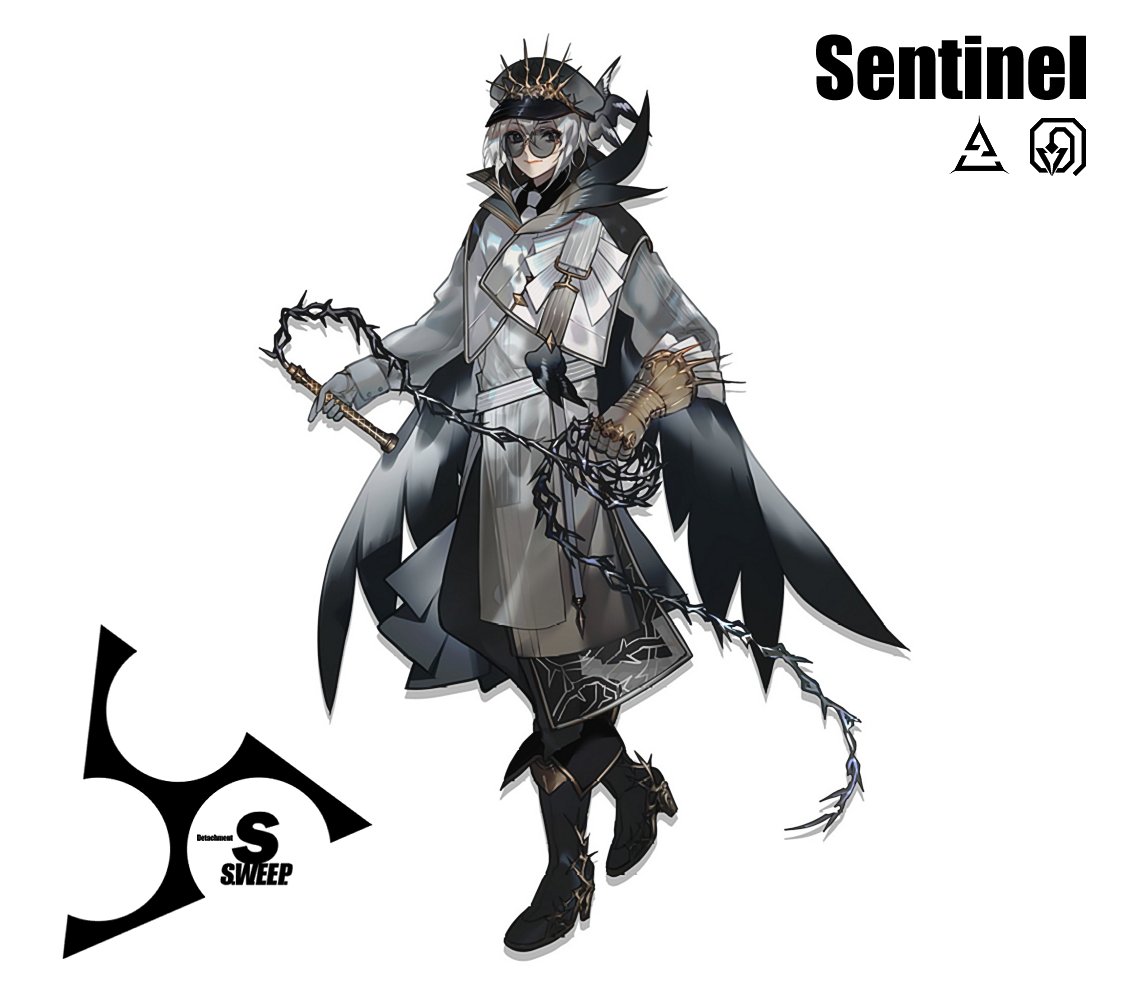The image features a detailed, anime-style character that exudes a villainous aura. The character, a woman, strides to the left on a clear white background. She is adorned in a gray metal jacket and black boots, both embellished with spikes. Her silver hair is partially concealed by a spiky black hat, reminiscent of a police cap with added pointy elements. Her eyes are hidden behind oversized, circular sunglasses. Black wings reminiscent of feathers or dark energy extend from her back. In one hand, she grips the handle of a barbed metal whip, which twists around her body and dangles to the ground, resembling a thorny vine. Her gloves are accentuated with dagger-like spikes. At the top of the image, the word "Sentinel" is prominently displayed in black font, accompanied by triangle and maze-like symbols with arrows. In the lower left corner, "S sweep" is inscribed, adding to the character's enigmatic presence. The overall impression evokes associations with Final Fantasy or Japanese role-playing games.